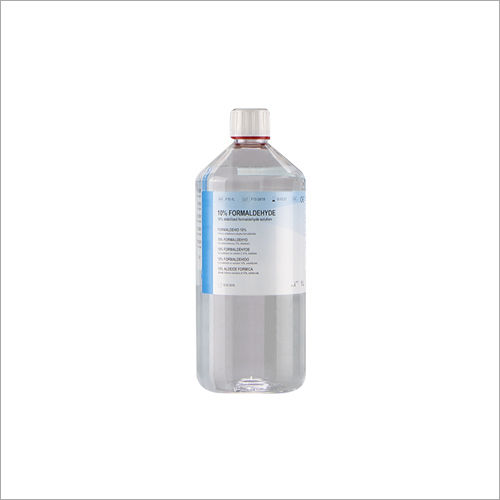The image features a large, shiny gray plastic bottle of chemical solution set against a white background. The bottle has a stout, round body and is topped with a shiny white cap that features vertical lines. A distinctive red ring encircles the base of the cap. The center section of the bottle is adorned with a label that wraps around its circumference. This label is predominantly white with a thick blue vertical stripe on the left side. The upper part of the label is pale blue, transitioning to a lighter blue at the bottom. The text on the label includes "10% Formaldehyde" in black, bold letters, with the word "Rebirth" written below. Additional smaller text is present but not legible from the image. The bottle also exhibits a textured indent or potential damage near the bottom center. The overall composition underscores the bottle's chemical contents and detailed labeling.